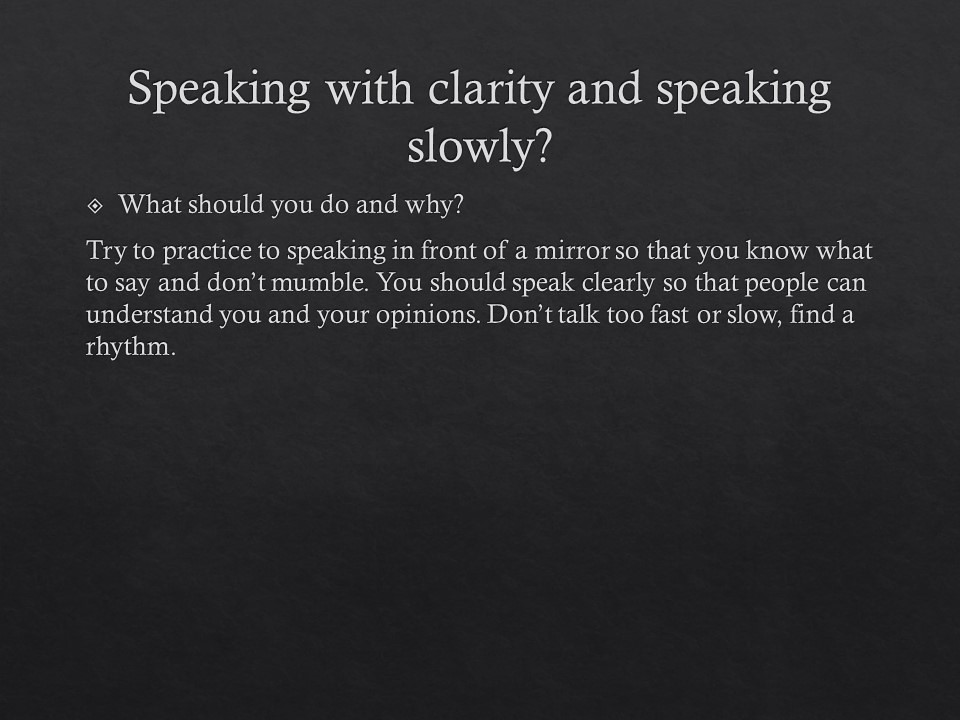The image is a rectangular design, oriented horizontally with a black background. The top half of the image features bold, white text. At the center, in large letters, it reads "Speaking with Clarity and Speaking Slowly," with "Slowly" positioned directly beneath "Clarity." Below this main header, aligned to the left but still positioned in the upper half, is a small white diamond bullet point followed by the text, "What should you do and why?"

Beneath this question, there is a paragraph of advice written in smaller white print, spanning four lines without indentation. It reads: "Try to practice speaking in front of a mirror so that you know what to say and don't mumble. You should speak clearly so that people can understand you and your opinions. Don't talk too fast or slow. Find a rhythm." The bottom half of the image is entirely plain, a void of blackness adding to the stark contrast and emphasis on the instructional text above.